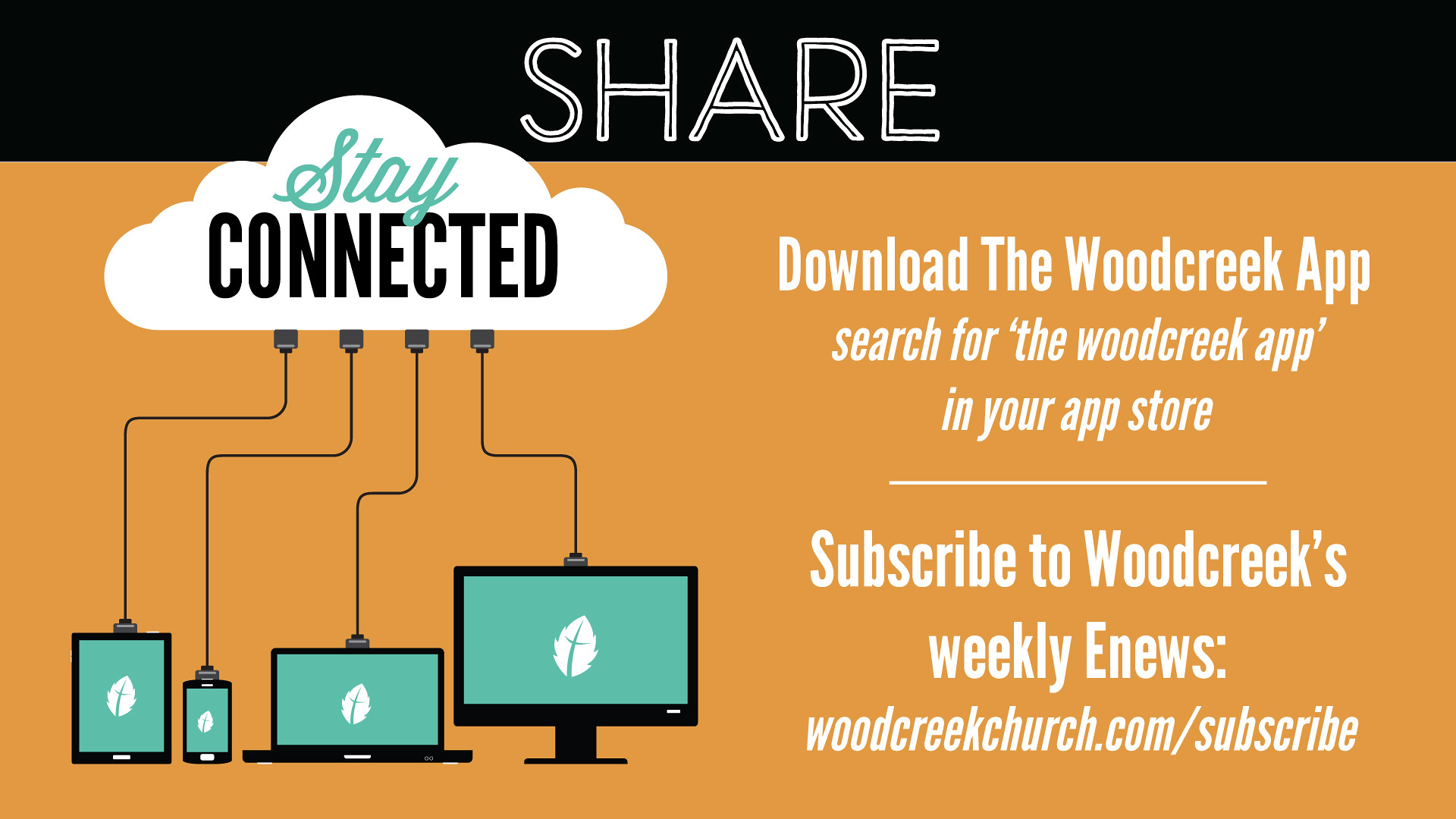The advertisement image features a burnt orange background with a prominent black banner at the top displaying the word "SHARE" in bold white letters. On the left side of the graphic is a cloud illustration with the words "STAY CONNECTED." The word "STAY" is styled in blue cursive font while "CONNECTED" is in bold black letters. From the cloud, four wires extend downwards, each connecting to different devices including a tablet, cell phone, laptop, and desktop computer. Each screen displays a green background with a small leaf logo featuring a cross. On the right side, the text in white font instructs viewers to "Download the Woodcreek App," and "Search for the Woodcreek app in your app store." It also encourages them to subscribe to Woodcreek's weekly e-news at "woodcreekchurch.com/subscribe." The overall design serves as an infographic, promoting the Woodcreek church app and newsletter subscriptions.